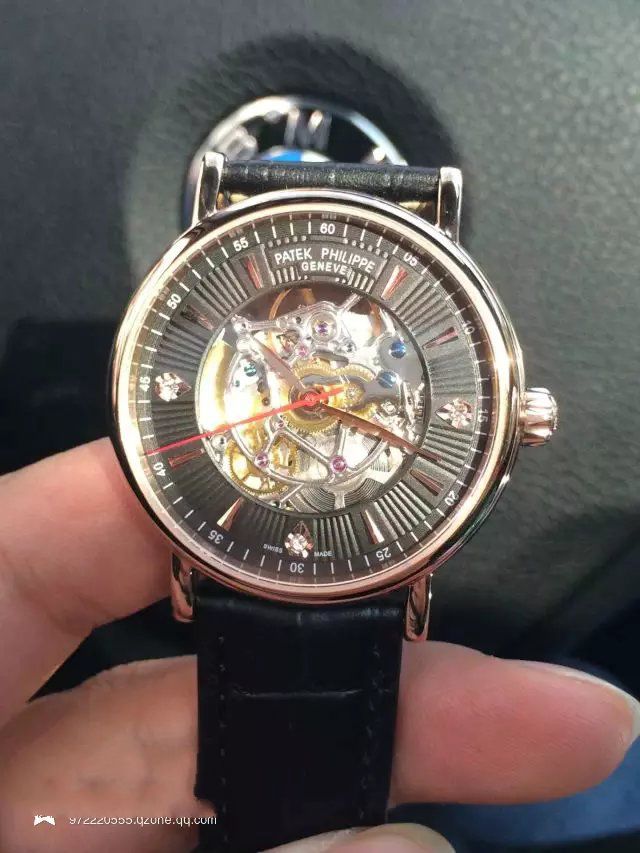This photograph features a luxurious Patek Philippe analog wristwatch, meticulously crafted in Geneva and exemplifying Swiss precision as proudly indicated on the dial. The watch boasts an elegant black face, which intriguingly reveals the intricate inner clockworks at its center. Complementing its sophisticated design, the hour and minute hands, along with the surrounding bezel and dial, are rendered in a gleaming gold hue. The exquisite timepiece is strapped onto a black leather band.

In the foreground, the watch is delicately held by a woman whose well-manicured fingers enhance the elegance of the shot. The setting of the photograph is brightly lit, capturing fine details that suggest the image was taken inside a vehicle. The background subtly includes the black dashboard and a faint glimpse of a BMW emblem, situating the scene within a car. Notably, there is some form of writing in the bottom-left corner of the image, though it is not immediately identifiable as a date or any other specific detail.